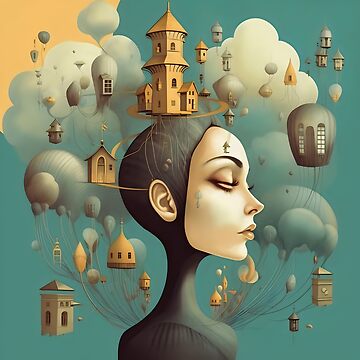The image is a vividly abstract, computer-generated scene with a distinct air of modern surrealism. The background is predominantly a teal green, transitioning into a blue-gray shade, with an eye-catching bright yellow sun or light source in the top left corner. Scattered white clouds add a whimsical touch to the sky. At the heart of the composition is a woman with exaggerated facial features, including prominent eyebrows, nose, and lips. Her eyes seem to be only slightly open, giving a dreamy, introspective appearance. The woman is dressed in a sleek, black catsuit-like garment that covers her neck and torso, leaving her ears exposed, and sports a distinctive pitchfork tattoo on her right jaw.

Surrounding her head and upper shoulders are numerous imaginative elements, possibly representing buildings, houses, and a clock tower. Some of these structures have an almost floating quality, with some resembling hot air balloons with windows and doors. There are also quirky walkways and roads connecting these structures to one another and to the woman, hinting at a fantastical, interconnected universe. The overall scene appears to be a fusion of realistic and fantastical elements, offset by the serene yet surreal background palette.